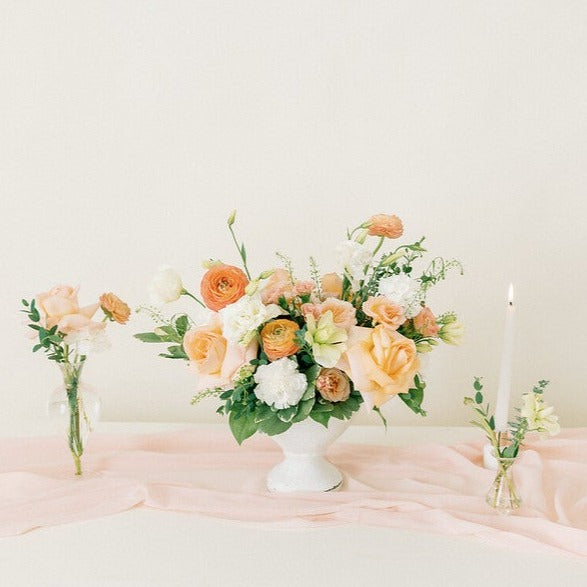The image depicts a serene and elegant table setting dominated by a pristine white backdrop. At the center of a white table draped with a light pink cloth, a large white ceramic vase holds a lush bouquet featuring a mix of dark orange, light salmon, blush pink, and white flowers, complemented by abundant green leaves. To the left, a small glass vase contains a trio of flowers — two light pink and one orange, with verdant stems. On the right, a tiny clear vase houses a single white flower accompanied by a few green leaves, positioned just in front of a lit white taper candle. The overall composition is aesthetically pleasing, with the soft hues and floral arrangements creating a harmonious and tranquil atmosphere.